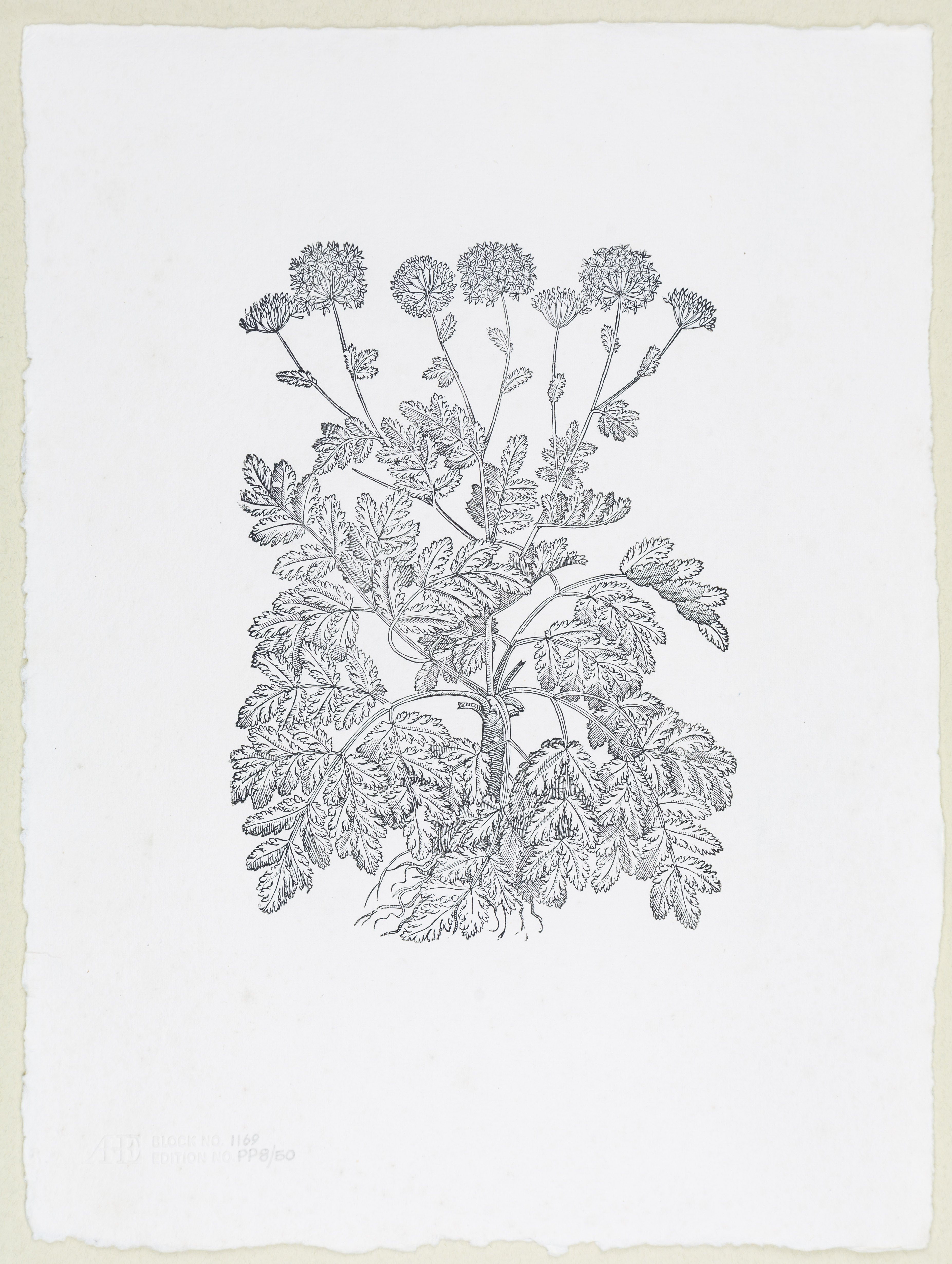This is a highly detailed black and white drawing of a plant with numerous leaves and flowers, made using black lines on a rectangular, white-colored surface, likely paper or canvas. The white surface is framed by a light, cream-colored or light wood-colored border. The drawing depicts a plant with compound leaves, each consisting of several leaflets, and is topped with around six to seven flowers, with four noticeably larger flower buds standing out at the top. The intricate and complex design captures the delicate beauty of the plant, although its black and white nature makes it challenging to identify the specific type of flower. The overall composition is set against a light lavender background, adding a subtle contrast to the monochromatic art.